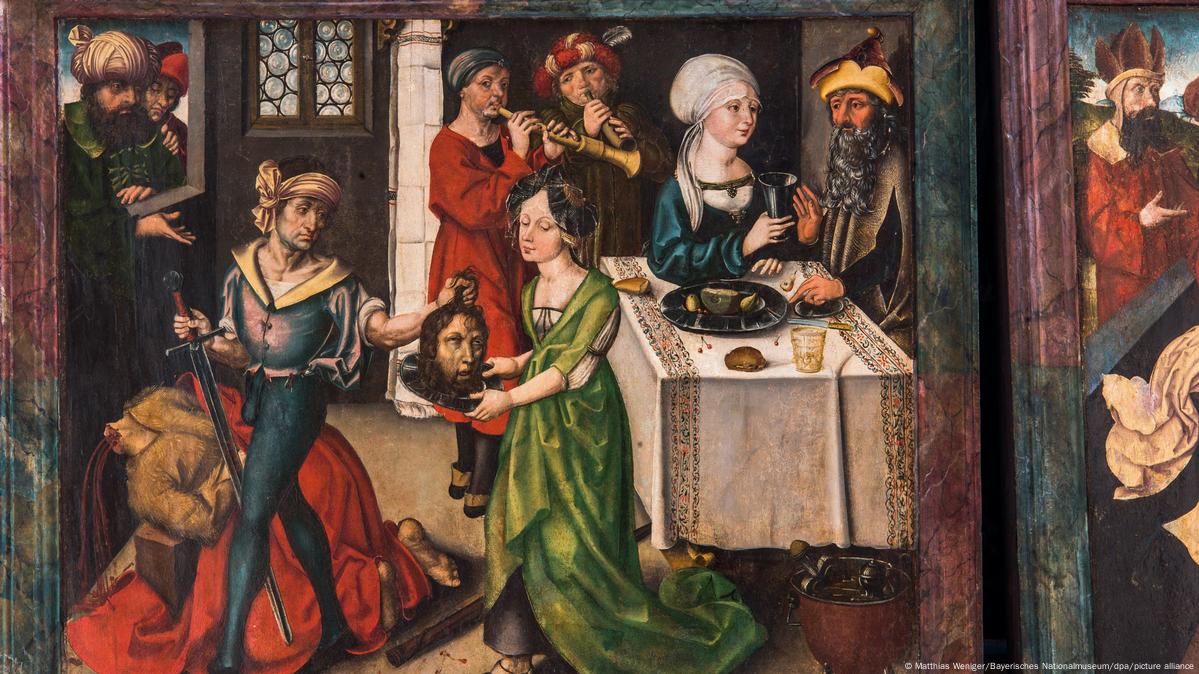This image, rectangular in shape and approximately six inches wide by three inches high, displays two framed paintings set side by side. Both paintings are housed in wooden frames painted in red with bluish gold accents. The painting on the left captures a vividly detailed, possibly medieval, indoor scene filled with various figures engaged in different activities. Starting from the right-hand side, a table adorned with a white tablecloth hosts two diners. To their left, two individuals play flutes. In front of them, a central and gruesome tableau unfolds: a man, potentially the focus of the painting and clad in black stockings, wields a sword as he decapitates another man, whose blood spills from his neck. The severed head is held by the man and is being admired by a woman in a green dress beside him. Lower left, the decapitated body is visible, lying on the ground. In the upper left corner, two onlookers gaze towards the macabre scene. The overall ambiance of the painting is dark, both in tone and content, despite the lively background activities of people playing instruments and enjoying food and drink. The adjacent painting on the right, mostly obscured, features a man in a red cloak and hat looking towards the right, implying continuity or contrast with the left painting's dramatic narrative.